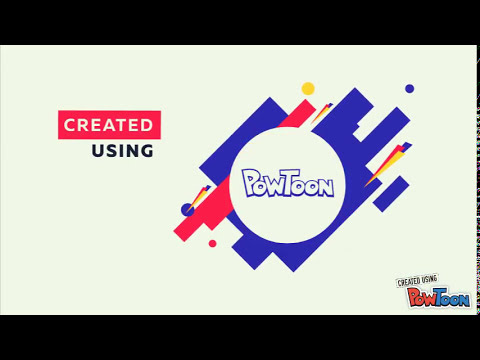This image is a detailed graphic design, likely the beginning of a video created using Powtoon. It features a wide rectangular layout with thick black bars across the top and bottom. The background is slightly off-white. In the upper left corner, there is a prominent red rectangle with the word "CREATED" in capitalized white font. Directly below, in bold black text, it says "using." On the right-hand side, there's a large white circle containing the word "Powtoon" in a cartoonish block font with a purple outline. Surrounding this circle are various diagonal rectangles in colors like blue, red, and purple, along with scattered triangles in yellow, pink, and purple, and smaller circles in red, blue, and purple. In the bottom right corner, the phrase "created using Powtoon" appears again, with "created using" in black text and "Pow" in a reddish color and "toon" in light blue.